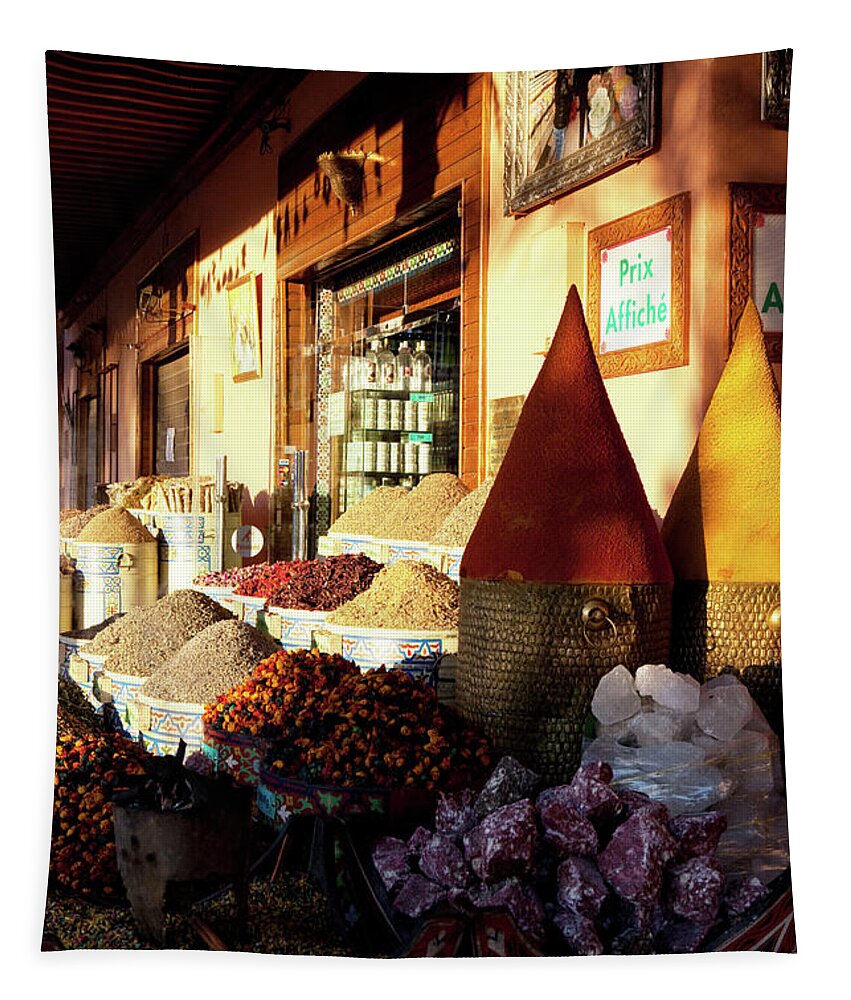The image depicts an outdoor scene of a storefront that appears to be in Europe, made evident by its sign displaying "Prix Afiche" in green text on a white background, though the exact language isn't identified. The store's façade features wood paneling above the door and possibly a brown awning. The sunlight illuminates the variety of natural items meticulously arranged in containers. Positioned in three rows, these baskets contain an assortment of grains and spices, with their typical beige hues prominently featured. To the right, two larger containers house yellow and red items, likely flowers. Among the vibrant display, there are striking orange dried flowers and various colored stones, including white, blue, clear, and reddish-purple rocks, contributing to the vibrant and multifaceted scene. The overall composition suggests a quaint, picturesque market setting perfect for capturing the essence of diverse, artisanal goods displayed in baskets and pots.